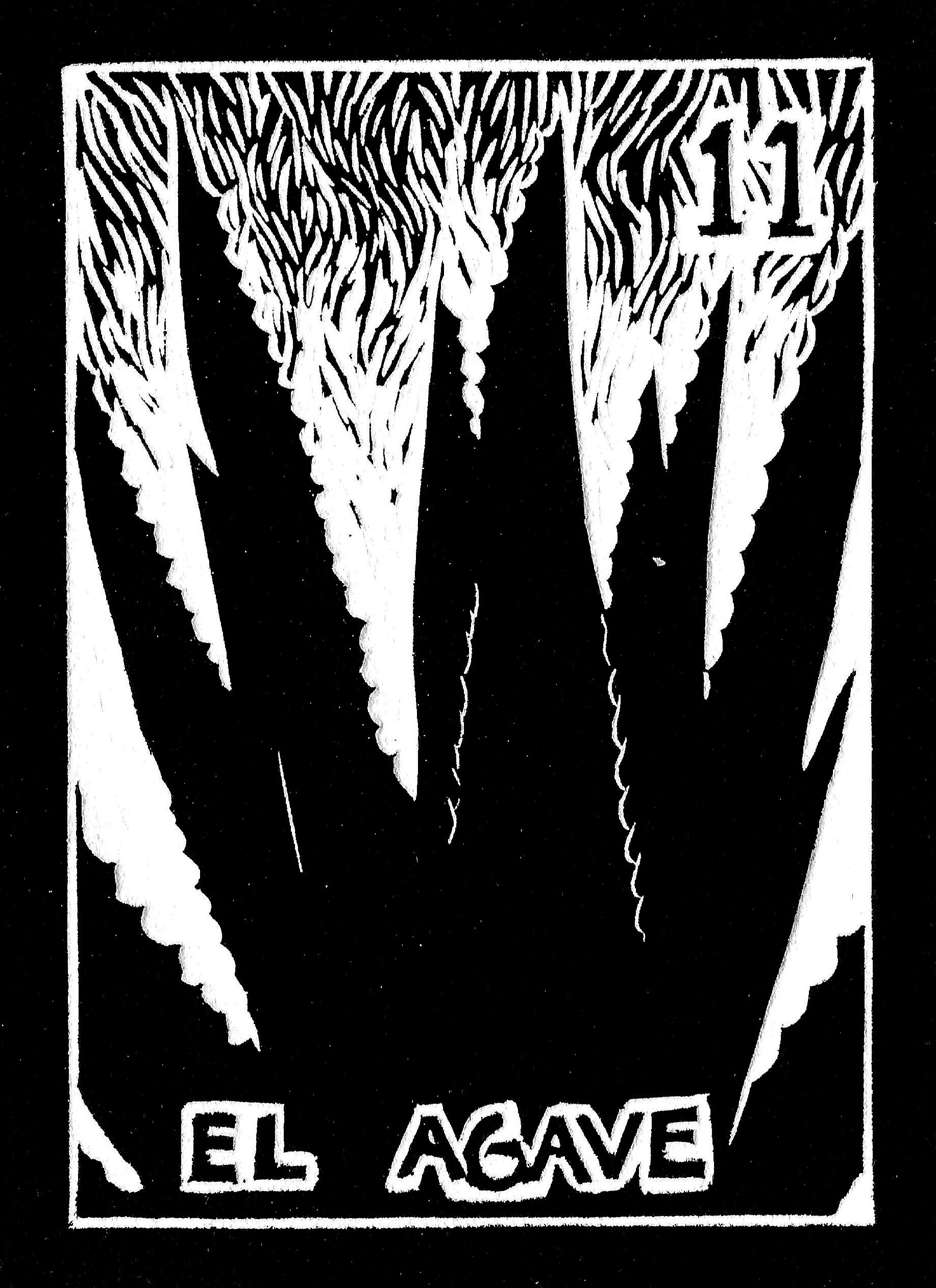The image is a detailed, black-and-white piece of art resembling a vintage trading card or playing card, prominently featuring an agave plant, which is known for being used to produce tequila and mezcal in Mexico. The artwork is rectangular with black borders. It displays the number 11 in the upper right corner while the words "EL AGAVE" are written at the bottom in bold, capital letters with a white border around them. The agave plant, depicted in negative space with jagged, needle-like tips on its leaves, stands out in black against a white background. Above the plant, there are intricate designs resembling tiny flames or lights, adding depth to the illustration.